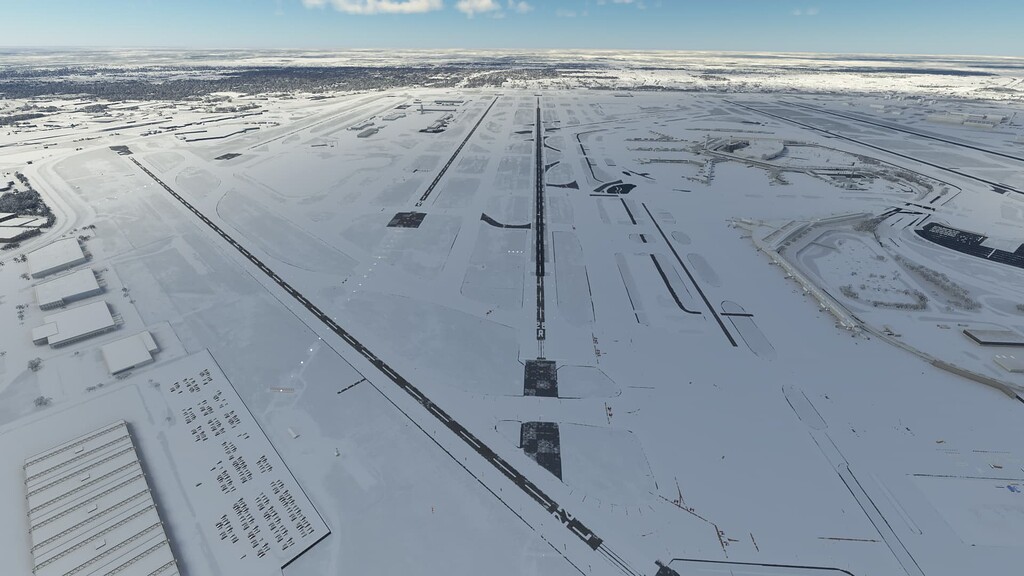This detailed, overhead photograph captures an expansive, snow-blanketed airport runway system, giving the illusion of a black and white image due to the contrasting white snow and dark runway lines. The central landing strip, flanked by two additional tracks on either side, extends towards a horizon dominated by a strikingly blue sky with a scattering of faint, puffy white clouds. The snow appears unevenly distributed, suggesting a heavier snowfall was previously cleared and now lightly re-dusted, revealing faint dark lines where the snow removal machinery passed. On the left side, the snow-covered tops of airport buildings or hangars are visible, mirrored by similar structures on the right. The scene is devoid of airplanes and people, emphasizing the serene, pristine winter landscape that stretches flat and uninterrupted to the horizon.